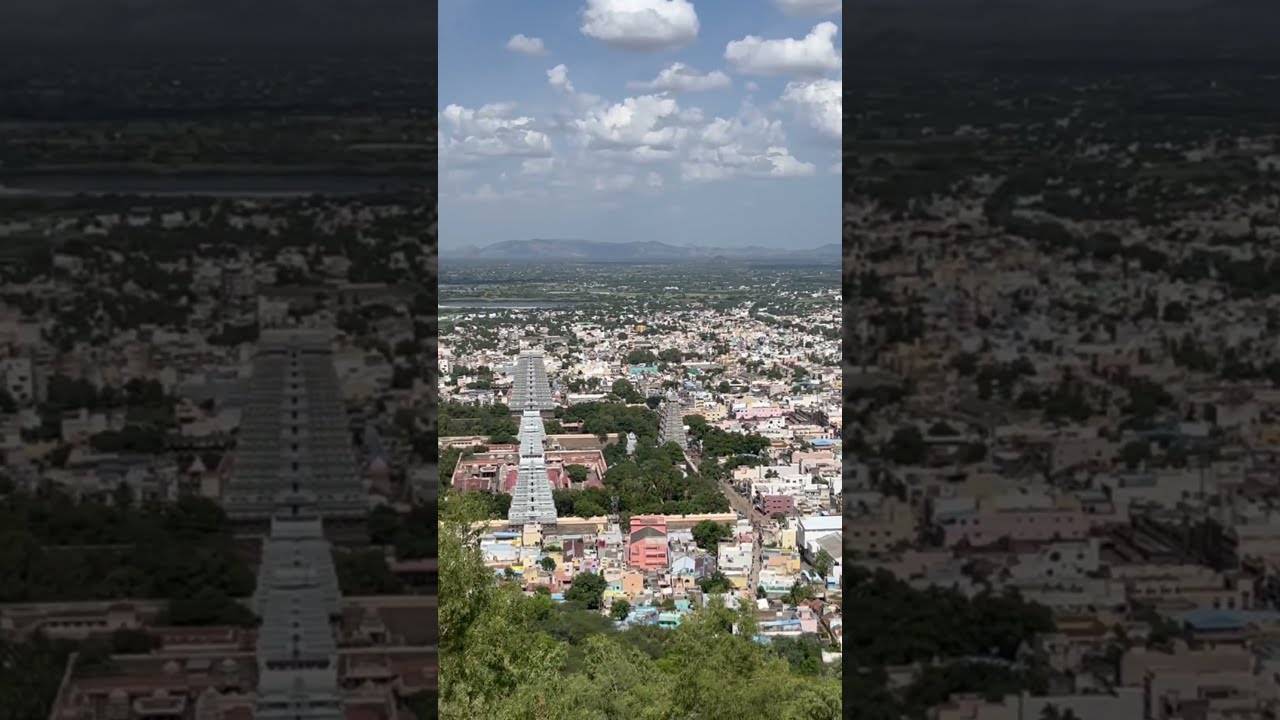This overhead photo captures a sprawling cityscape densely populated with numerous small, colorful buildings in shades of orange, yellow, and red, interspersed with patches of green trees throughout. The view extends towards a distant horizon where a serene body of water is partially visible on the left, leading further beyond to a majestic silhouette of mountains. Central to the image is an arrangement of taller towers and a large square courtyard or structure with more greenery within, providing a focal point among the sea of lower buildings. The sky above is a clear blue, adorned with scattered white clouds, and though the day appears sunny, there is a slight haze suggesting mild smog or fog. The city stretches widely, seamlessly integrating built structures with natural elements, creating a vibrant and detailed urban landscape.